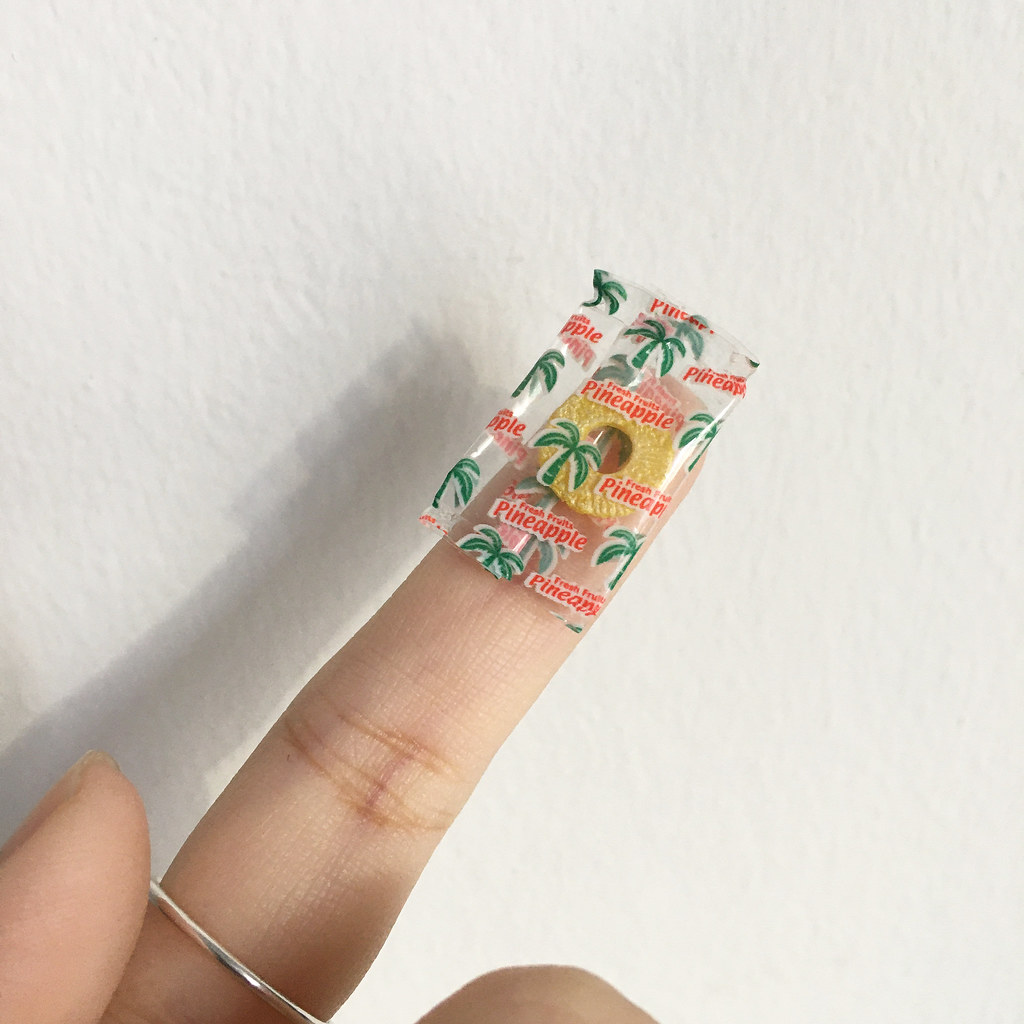A photograph captures a small, round, yellow candy, resembling a pineapple slice with a hole in the center, wrapped in a clear package adorned with little green palm trees and red text reading "Fresh Fruits Pineapple." The candy is balanced on the tip of a Caucasian left hand's index finger, which is notably adorned with a thin silver ring. The thumb and part of the middle finger are curled around the palm, with the short fingernail of the thumb slightly visible. The background is a textured white wall, casting a long shadow of the finger and candy package, emphasizing the detailed features of the scene.